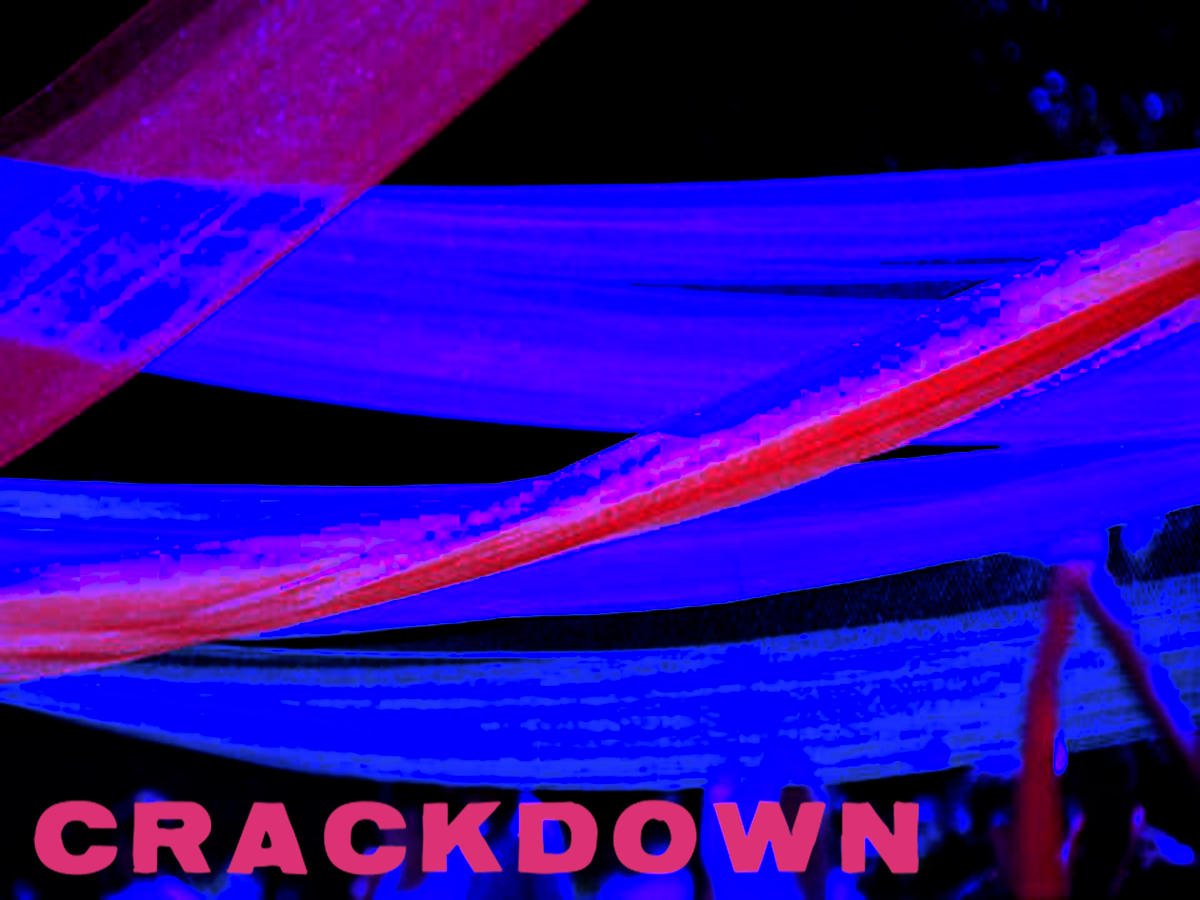The image is a highly abstract, posterized piece with minimal color variation, featuring bold, psychedelic colors against a black background. Large, solid swaths of brilliant royal blue and vivid neon pinkish-purple (or fuchsia) streak diagonally across the frame. At the bottom, in all capital letters, the word "CRACKDOWN" is rendered in bright fuchsia text, standing out starkly. The overall aesthetic, characterized by its striking, vivid hues and abstract design, evokes a retro, 60s album cover vibe, possibly created using Photoshop to enhance the eye-catching psychedelic effect.